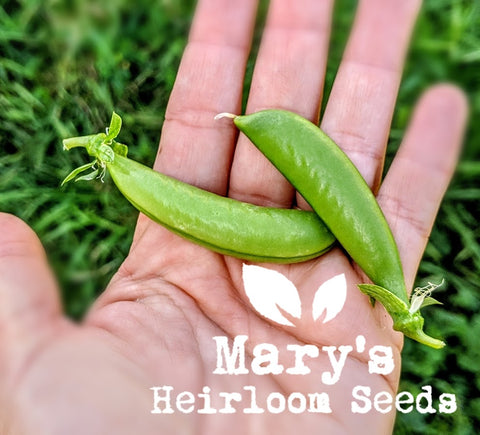A square photograph features the left hand of a white person, palm facing up, with detailed lines visible on the skin. Resting in the palm are two small green pea pods, each about the size of the person’s pinky finger, with cut stems at the ends. The background consists of slightly blurry, lush green grass, adding a vibrant, natural setting. Positioned in bold white font in the bottom right corner, the text reads "Mary's Heirloom Seeds," accompanied by two white oval-shaped leaves as part of Mary's logo. This adds a professional touch, indicating the image likely serves as an advertisement for Mary's heirloom seed business.